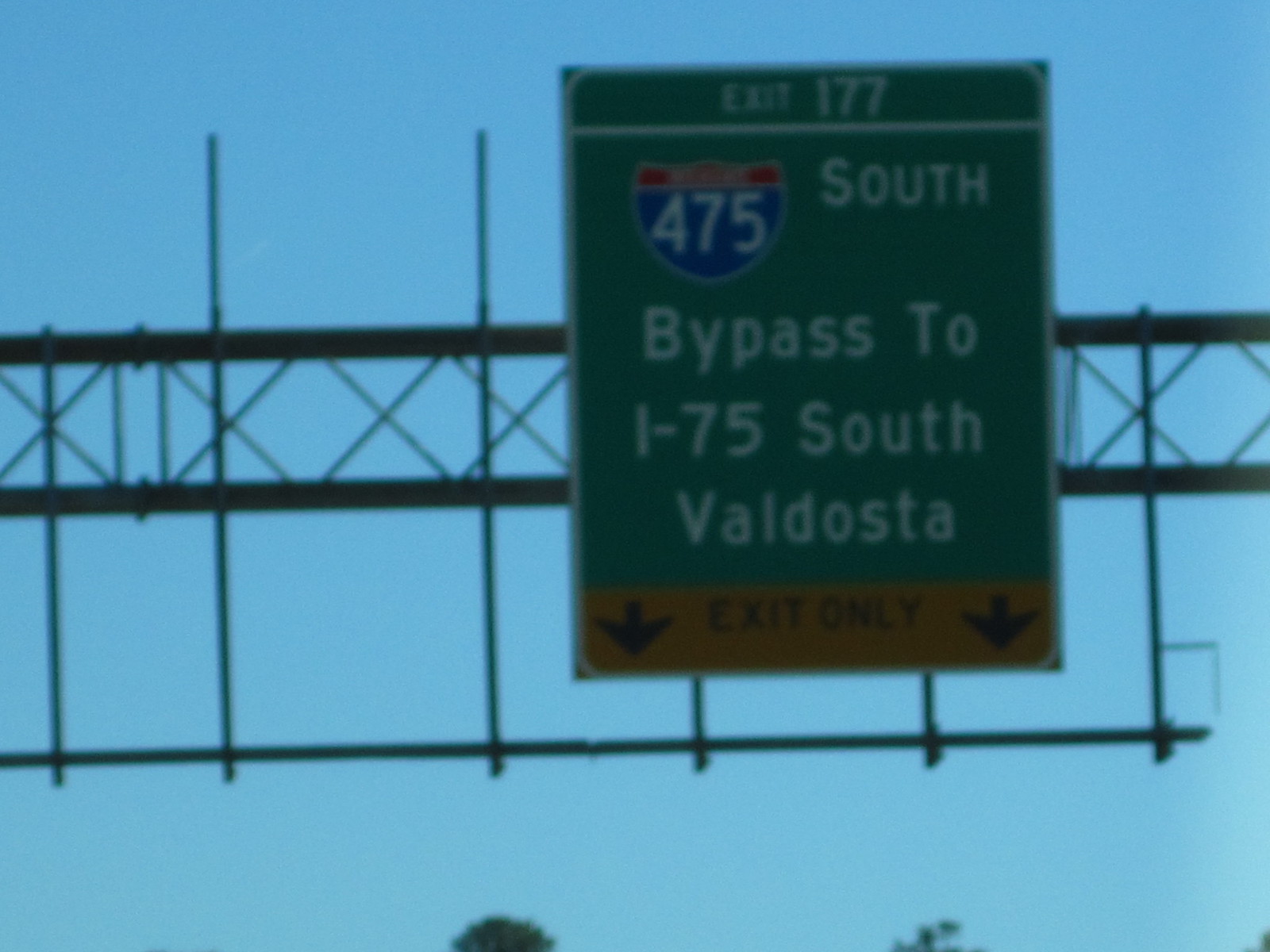The image captures a scene on an American freeway, taken from a moving vehicle. The focal point is a somewhat blurry, zoomed-in road sign suspended over the highway. The green sign indicates Exit 177 on I-475 South, directing drivers to a bypass leading to I-75 South towards the city of Valdosta. The sign is mounted on a metal gantry, which spans across the wide freeway, offering clear instructions for motorists. The overall impression is one of motion, with the out-of-focus quality hinting at the speed of travel and the dynamic nature of freeway driving.